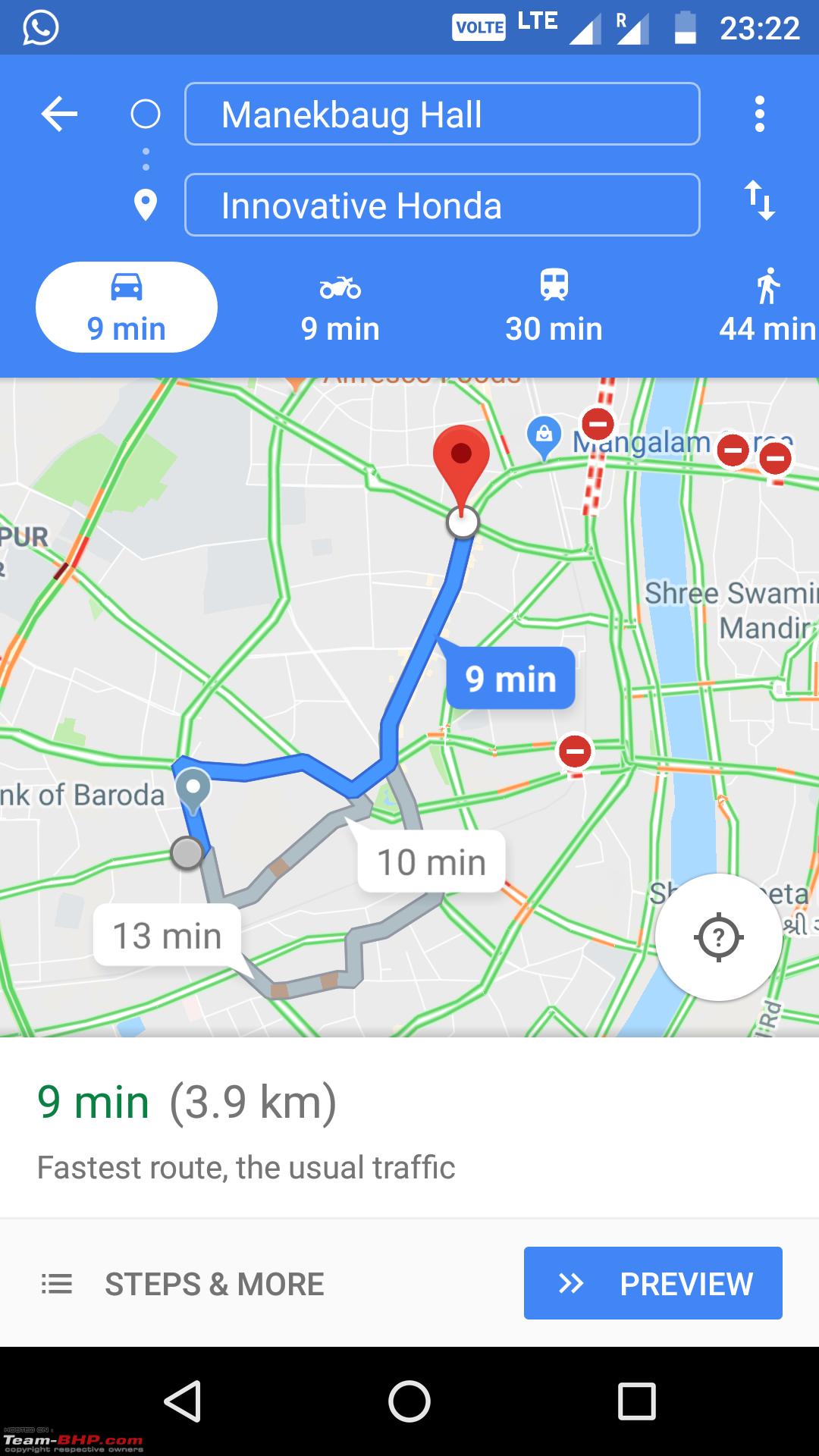Here is a cleaned-up and detailed caption for the image described:

---

**Screenshot of a Map Interface: Detailed Description**

In the center of the image is a map focusing on various pathways. The primary route, highlighted in green, is marked with a time of nine minutes. There are several chat bubbles pointing towards different segments of the map: one at the nine-minute mark indicates a blue pathway, another at ten minutes points to a gray path, and a third at thirteen minutes highlights another section of the gray path. Red circle markers with minuses in them (four in total) appear: three in the upper right-hand corner and one in the middle-right portion of the map. A stream or body of water is visible on the right side, colored blue. At the top left of the image, there are phone UI icons including a chat bubble, LTE symbol with text "VoLTE," the time "23:22," battery usage indicator, and Wi-Fi status.

Below these UI icons, there is a search bar displaying “Minic Bog Hole” with three dots on the right. Another search bar below it reads “Innovative Honda,” accompanied by a blue icon featuring two arrows pointing up and down. Next to this search bar is a white marker icon. Additionally, a white tab displays transportation modes and times: a car (nine minutes), bike (nine minutes), bus (thirty minutes), and walking (forty minutes). The map also shows a route description: "Nine minutes (3.9 km)" in green text, with "Fastest route, usual traffic" beneath it in gray. There is an option labeled "Steps & More" next to a "Preview" button, featuring two arrows pointing left and right.

At the bottom of the map, a black bar contains triangular, circular, and square icons. Text in small white and red font appears in the lower left-hand corner.

---

This caption provides a detailed, organized, and comprehensive description of the various elements in the screenshot.